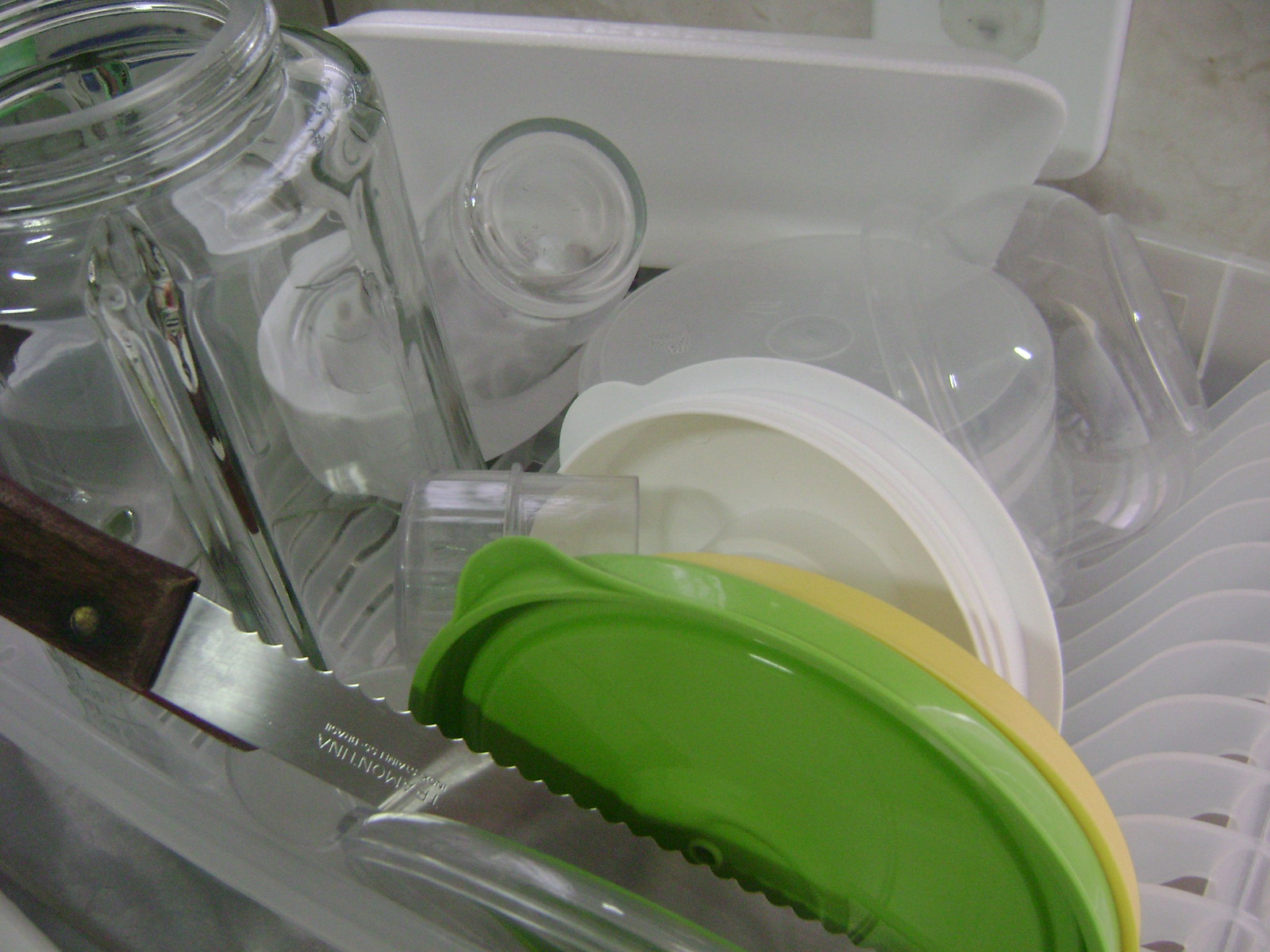In the image, a white plastic dish-drying rack is positioned against a white marble backsplash. The translucent, whitish rack is filled with various kitchen items. On the left side, there is a clear, empty, square glass jar with slightly rounded edges at the top. Next to the jar, a serrated knife with a brown handle and a long silver blade rests precariously. Scattered throughout the rack are various plastic container lids, including a green circular one, a yellow circular one, and a smaller white circular one. Additionally, there is an upside-down small plastic bowl and an upside-down glass nestled inside it. A thick, white plastic lid, possibly the matching lid for the glass jar, is also present. Further adding to the assortment is an upside-down cylindrical plastic container and a white plastic serving tray, both drying alongside the other items in the rack.